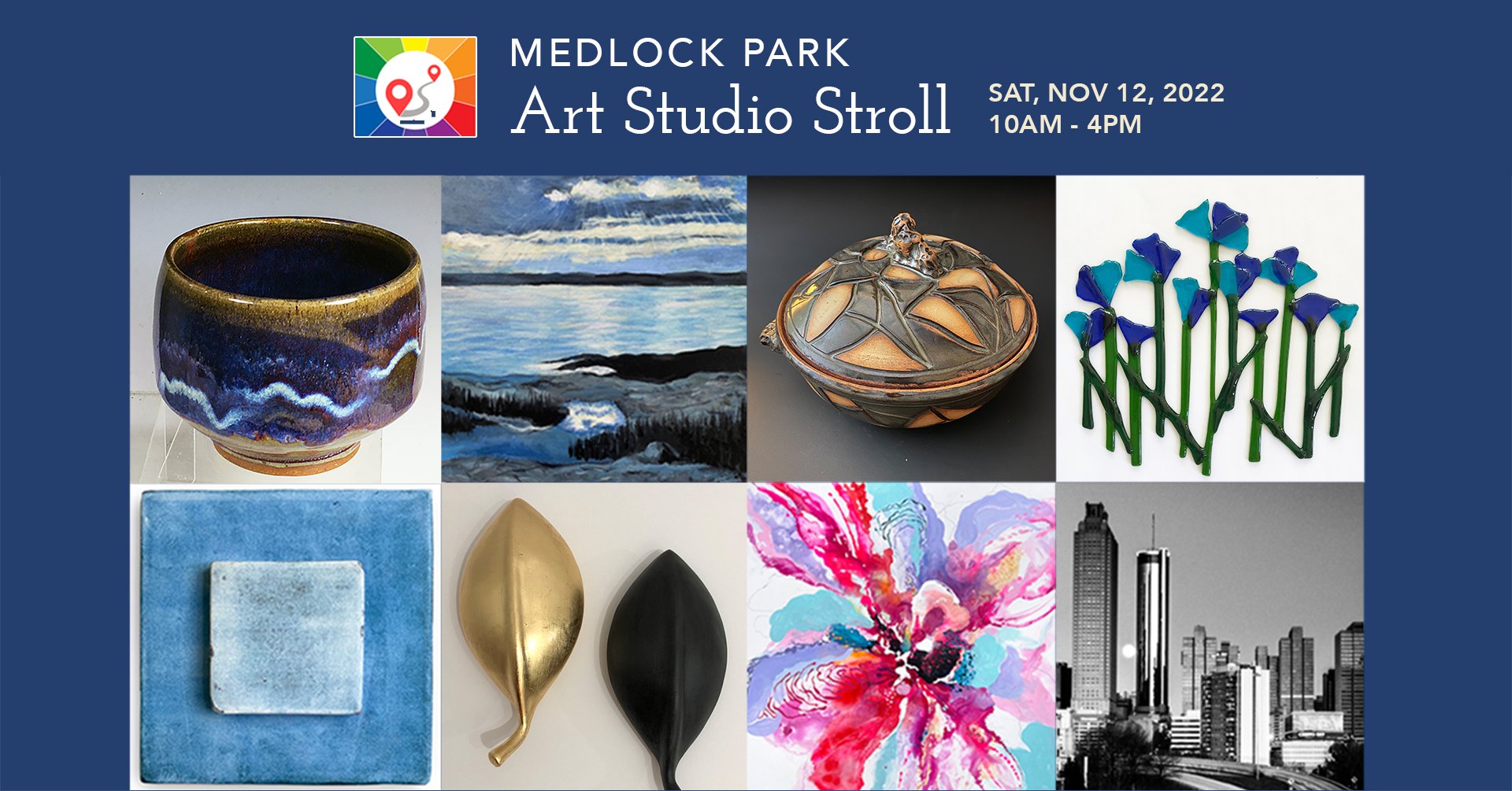The image is an advertisement for the upcoming "Medlock Park Art Studio Stroll" event, scheduled for Saturday, November 12, 2022, from 10 a.m. to 4 p.m. The advertisement is presented in landscape mode with a blue background and prominently features a white circle icon with two red location markers surrounded by rainbow-colored rays. Below this icon, the event details are printed in clear text.

The advertisement showcases eight images representing various artworks that will be featured at the event. The top row includes:
1. A tan and blue ceramic bowl with white stripes.
2. An oil painting depicting an ocean scene with crashing waves and an overcast sky.
3. An orange and brown pottery piece with a lid.
4. A glass art piece with blue flowers on green stems.

The second row features:
1. A ceramic tile with golden and black leaves.
2. A vibrant, multicolored floral painting.
3. A black and white photograph of a cityscape.
4. Artwork that could either be watercolor or metal art, comprising intricate designs with gold and black leaves.

This detailed collection highlights the diverse range of artistic expressions that attendees can expect to explore at the Medlock Park Art Studio Stroll.